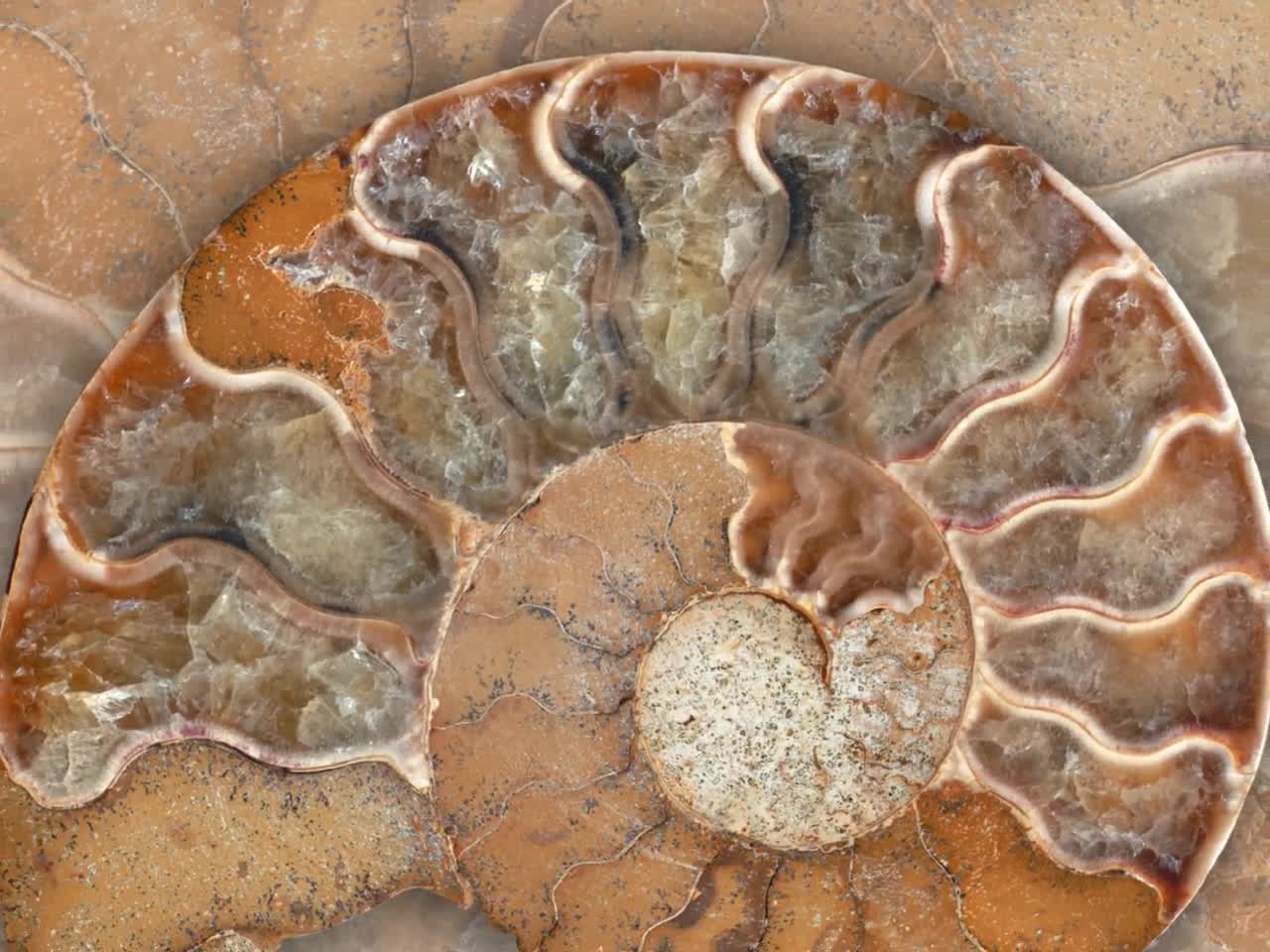The image depicts a broken ceramic plate resting on a russet brown tile, which features distinct lines running through it. The plate, fragmented and incomplete, showcases a color palette of brown, orange, and russet with notable white outlines in its pattern. The broken ceramic pieces, missing in parts, give the appearance of a snail or the shell of a shrimp, curling into a semicircle at the center. The russet brown tile underneath adds to the overall texture with its granite or stone-like quality, highlighted by flecks of brown and white. The plate's design is further accentuated by a white border and intricate, squiggly lines creating inlets that traverse across its surface. The interplay of colors and shapes evokes a sense of curiosity and natural form, blending man-made artistry with elements reminiscent of nature.